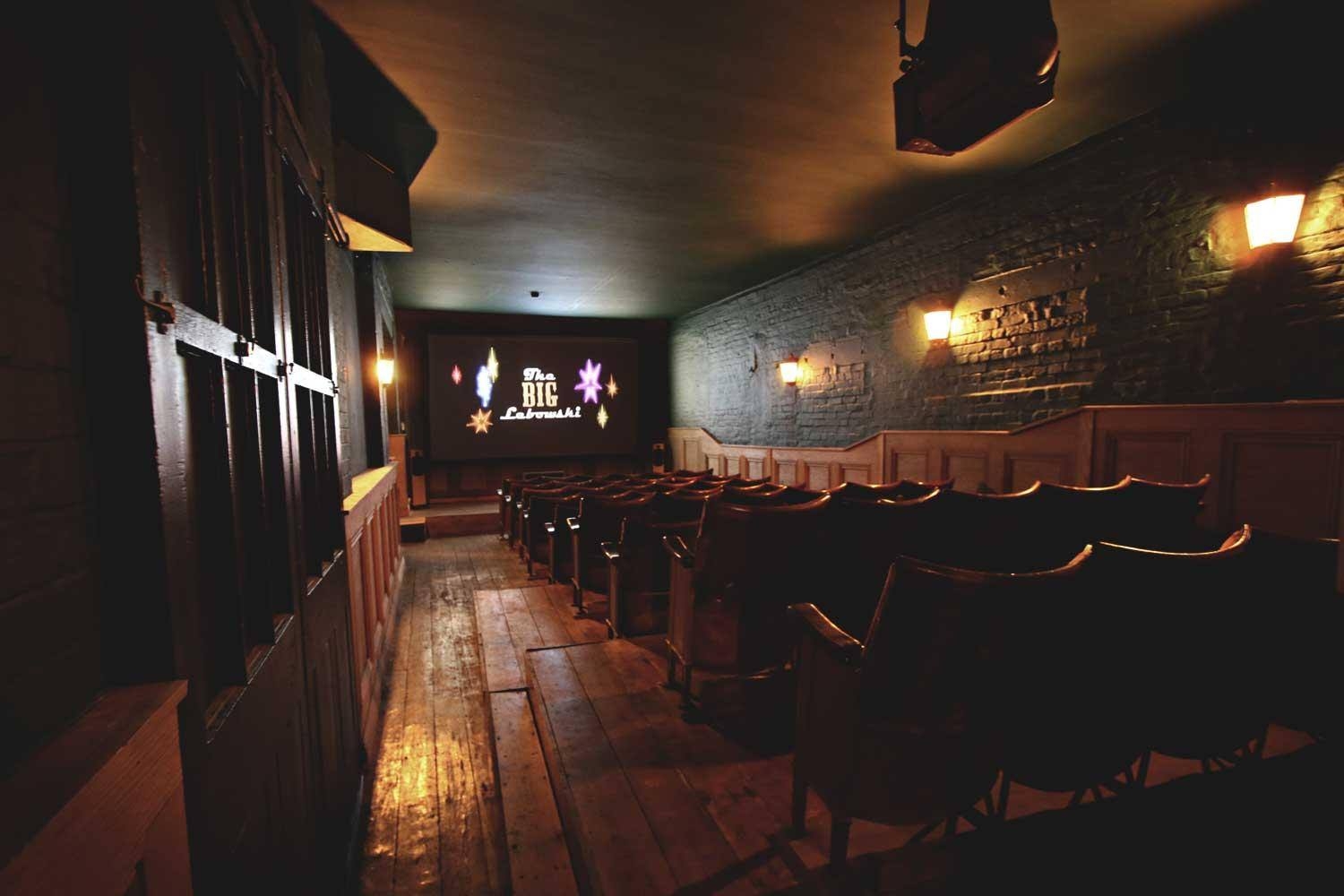This photograph captures a charming, old-style private theater, likely nestled within someone's home. The theater boasts seven rows of seating, with each row containing between two to five brown seats, arranged in a narrow formation for an intimate viewing experience. The flooring consists of vintage-looking hardwood floorboards that slope downward towards the screen, indicative of stadium seating. 

On the far side of the room, a black screen displays a scene from "The Big Lebowski." Above, the film projector is visibly suspended from the ceiling. The walls of the theater add to its rustic charm: the left wall is painted green on top, transitioning to tan wainscoting at the bottom, and is adorned with four sconce lights as well as wooden cabinets. The right wall features a combination of brickwork on the upper half and wooden boards on the lower half, complemented by wooden shelving units.

Overall, the theater's decor, including green walls, tan wainscoting, and intricate wooden elements, evokes an old-fashioned and cozy atmosphere, reflecting a bygone era of cinema.